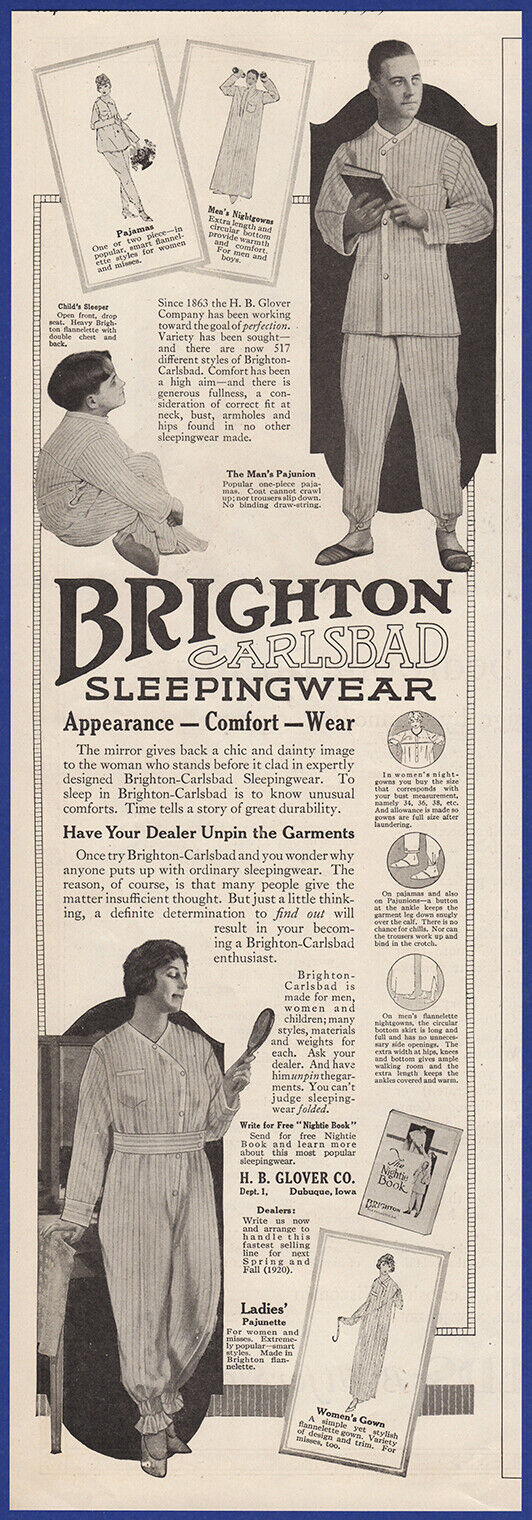This monochromatic illustration, reminiscent of a 1950s newspaper advertisement, prominently titles "Brighton, Carlsbad Sleepingwear." It showcases various figures - a man, a child, and a woman - all clad in striped, practical, button-down pajamas. The central figure, a man, stands at the top holding a book, gazing forward. To his left, a young boy sits on the floor, looking up at him. The bottom portion features a woman stepping near a wardrobe, holding a mirror. The woman is dressed in a slightly more feminine version of the sleepwear, and another drawing of a woman in a gown is also present near her. The advertisement, bordered in blue, is styled as a thin vertical rectangle filled with black and white illustrations. Additional text phrases such as "Appearance, Comfort, Wear" emphasize the practical and comfortable nature of the sleepwear being advertised.